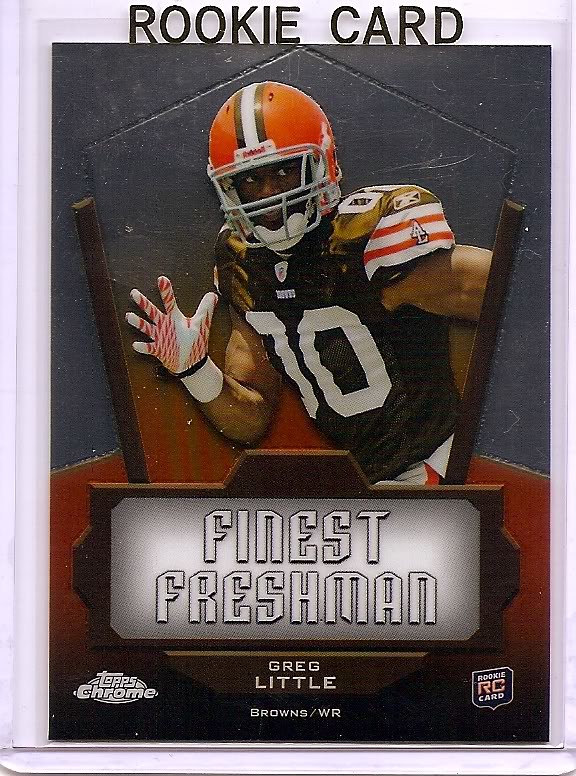In this image, we have a detailed trading card featuring Cleveland Browns wide receiver Greg Little. The card, which takes up the entire photo and is surrounded by a white border, prominently displays the words "Rookie Card" at the top and "Finest Freshman" at the bottom. The player, positioned centrally, is shown in full uniform with an orange helmet, a black jersey adorned with orange and white stripes on the shoulders, and matching orange and white gloves. Greg Little's name and his team affiliation, the Cleveland Browns, are also clearly indicated. He appears to be in motion, possibly running to catch the ball, with his shoulders arched back and looking towards the camera. The card features the Top’s Chrome logo and includes logos in the lower left and right corners, though the fine print details can be hard to discern. The background showcases dark, varying shades of gray, creating a pentagon shape that adds depth to the card, making it a collectible item likely cherished by fans and collectors alike.